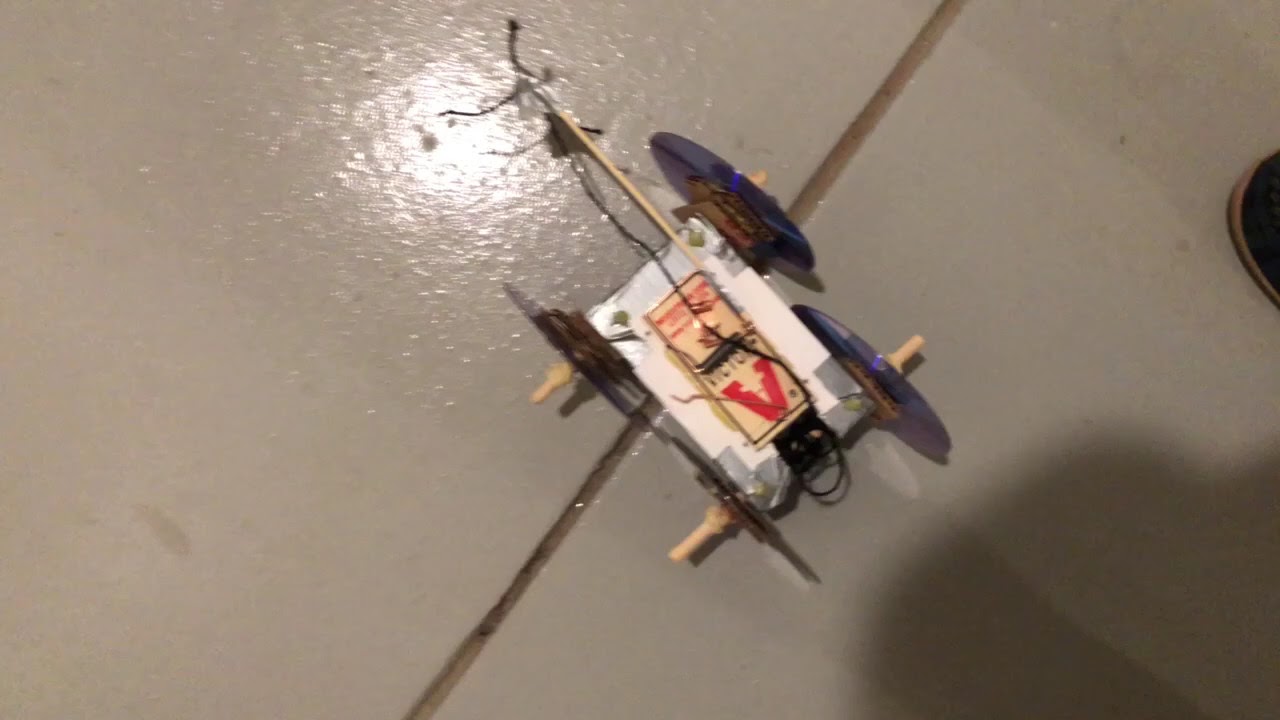The image shows a white, textured, tiled floor with a diagonal grout line running from the bottom to the top. Placed in the center of the image is a homemade contraption that features a white rectangular base. This base has wooden pegs protruding from each end, functioning as axles with silver, shiny CDs mounted on them to act as wheels. On top of this rectangular base, there is a small rectangular mousetrap with a noticeable red letter and a black lever across it. To the far right of the picture, partially visible, is a shoe with a brown sole and a navy blue or black upper. The setting is seemingly indoors, possibly someone’s home, and the overall appearance suggests a creative, improvised setup.